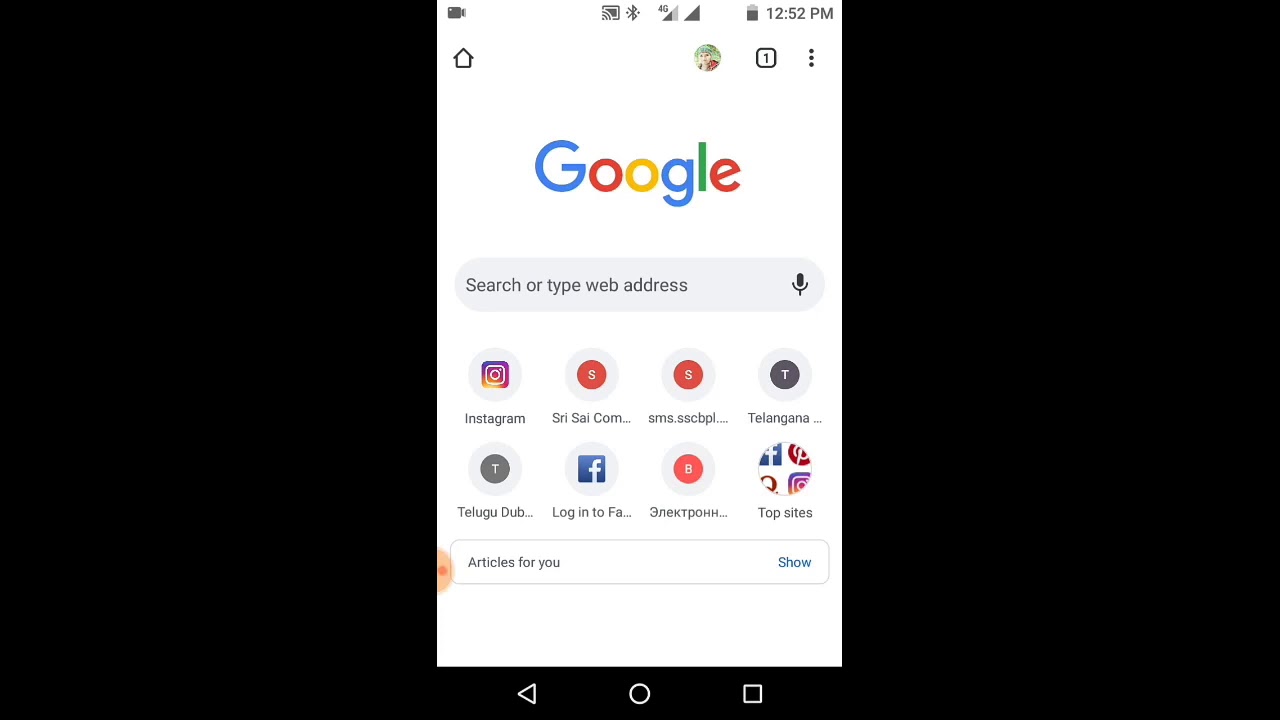A detailed descriptive caption for the given image could be:

---
The image displays a digital screenshot embedded within a black rectangle, showcasing the Google homepage. In the top left corner, an icon resembling a video camera is visible. Adjacent to it, a computer monitor icon appears, which includes symbols indicating a Wi-Fi signal in the bottom left, a Bluetooth signal, a 4G network connection with bars half-filled, and another connection with fully filled bars. The current time reads 12:52 PM, and the battery icon shows it is 75% charged.

On the left-hand side of the screenshot, there is an icon depicting a house, while the right-hand side features a person's avatar. Underneath this avatar, there is a square marked with the number "1" and a vertical stack of three ellipses.

Centered on the page, Google’s logo is prominently displayed in blue (G), red (O), yellow (O), blue (G), green (L), and red (E) on a white background. Beneath the logo, a gray oval search bar contains the text "Search or type web address" and a black microphone icon for voice input.

Below the search bar, there are eight icons representing different applications and sites: 
1. Instagram’s camera icon in purple and yellow within a gray circle.
2. An app abbreviated as "shreesicom..." within a gray circle with an orange inner circle and the gray letter "S" at its center.
3. "SMS dot SSCBPL..." with the same icon as shreesicom.
4. "Telangana..." in a gray circle enclosing a slightly darker gray circle with a white "T."
5. "Telugu dub..." in a gray circle, lighter than Telangana’s, with a white "T."
6. "Log into Facebook," partly visible with "FA..." in a blue square and a white "F."
7. An app with Cyrillic characters, displayed in a gray circle with an orange inner circle and a white "B" in the center.
8. "Top Sites," partially showing icons for Pinterest, Facebook, Quora, and Instagram within a cut-off gray circle.

Additional text "Articles for You" appears near an interactive text box with a "Show" button next to it. The rest of the screen is mostly white space. On the left edge, an orange dot with a semicircle extends partially into the screen’s frame, its purpose unclear.

At the bottom of the screenshot, traditional navigation symbols are present: a left-pointing triangle, a circle, and a square aligned horizontally.
---

This detailed caption closely describes each visual element in the screenshot, providing a clear and comprehensive understanding of the image contents.